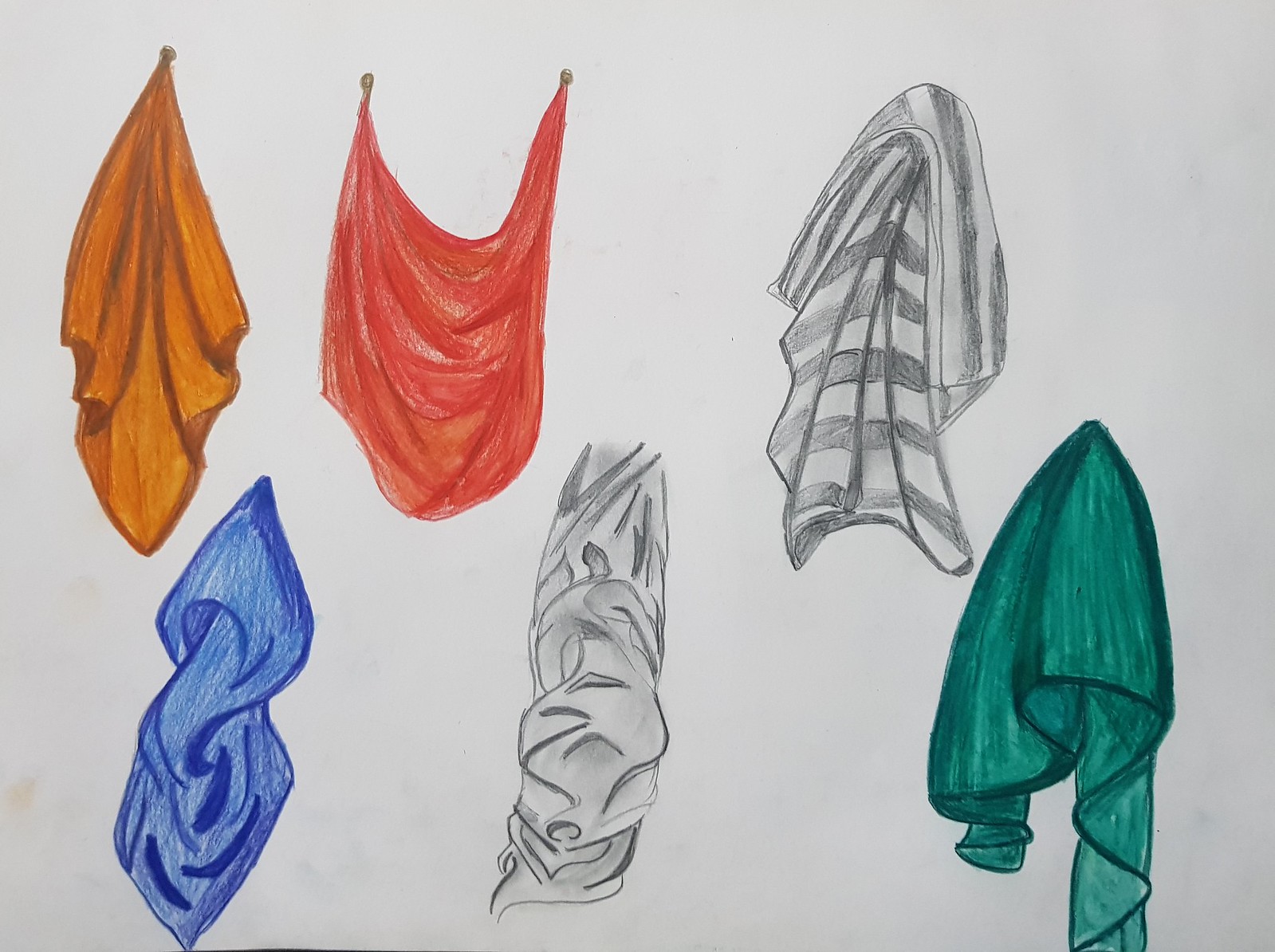This illustration features a collection of fabrics, each rendered in colored pencil, set against a pristine white background. In the top left corner, an orange piece of fabric is pinned to the wall, cascading down and folding slightly. Adjacent to it on the right is a red fabric, also pinned at the top left and right corners, spreading outward. To the extreme right, there is a white towel-like fabric adorned with black marks. Below, in the bottom left corner, lies a blue fabric, displaying visible folds. Centrally located, another fabric is present, primarily white with touches of gray and faint folds. Finally, to the far right, a green scarf is pinned in an elegant drape. Throughout the composition, the fabrics are lightly colored, with darker shadings accentuating the folds and giving depth to the illustration.